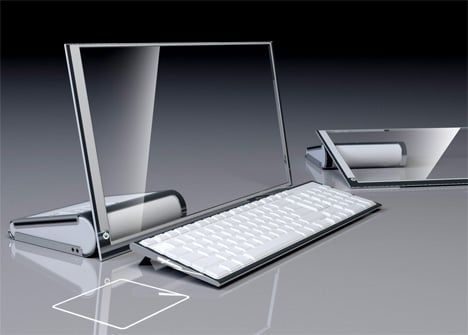The image depicts a futuristic concept for a projector monitor with a translucent screen, revealing the potential future of computer design. The main focus is a completely clear, glass-like monitor, supported by a stand behind it, ensuring it remains upright. In front of the monitor sits a sleek, white keyboard devoid of any lettering, emphasizing an advanced setup requiring familiarity with the key layout by touch. Positioned to the left of this keyboard is a clear square, possibly serving as a mouse pad or trackpad, which is usually found on the right. Additionally, another transparent screen can be observed to the right of the image, this one not propped up but resting on the stand. The reflective surface of the desk enhances the futuristic aesthetic by mirroring the combination of the screen and the stand.